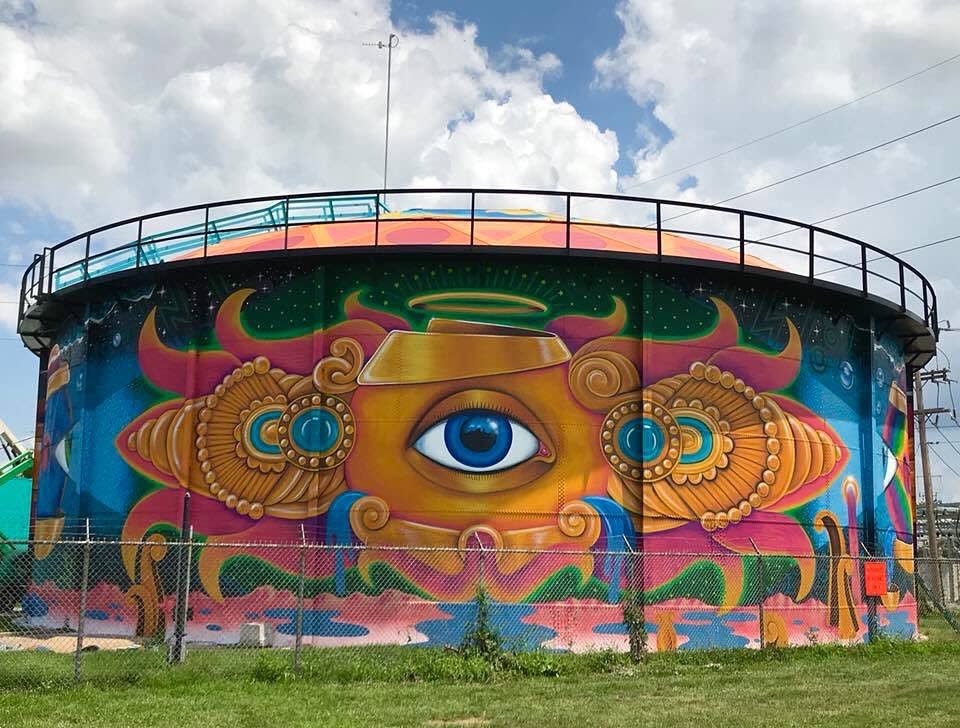The image captures a large, circular water tank positioned on the ground, not elevated in a tower. The tank features a vivid and surreal mural that dominates its visible side. The mural's focal point is a striking blue eye with a black pupil, surrounded by a golden crown-like structure adorned with blue jewel-like elements. This golden crown is topped by a halo. The eye itself is set against a backdrop that includes bright pink starburst effects, creating a vibrant contrast. The top and bottom parts of the eye integrate brown elements, resembling eyelids. Alongside the eye, the mural incorporates intricate details such as cornucopia shapes, water-like decorations, and various gold and blue circular motifs that enhance its ornate appearance. The structure appears to be positioned on closely-cut green grass, enclosed by a wire fence topped with barbed wire. In the background, the sky is a striking blue with large, white clouds, emphasizing the outdoor setting.